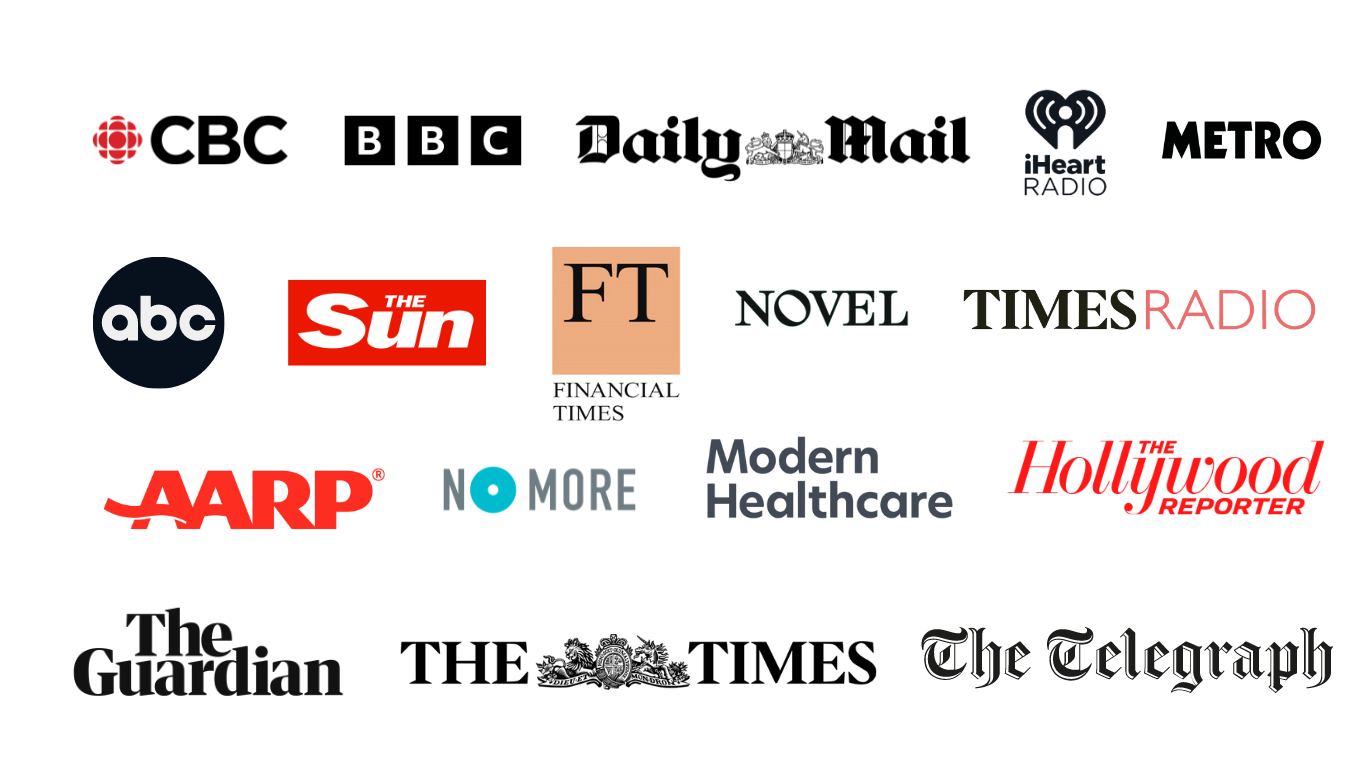This image showcases an array of company logos set against a plain white background, arranged in four horizontal rows from top to bottom. 

In the first row, from left to right, we have: 
1. CBC 
2. BBC
3. Daily Mail
4. iHeartRadio
5. Metro

In the second row, from left to right, the logos displayed are:
1. ABC
2. The Sun
3. Financial Times
4. NPR
5. Times Radio

The third row features, from left to right:
1. AARP
2. No More
3. Modern Healthcare
4. The Hollywood Reporter

In the fourth and final row, from left to right, the logos are:
1. The Guardian
2. The Times (with unique black and white artwork between "The" and "Times")
3. The Telegraph